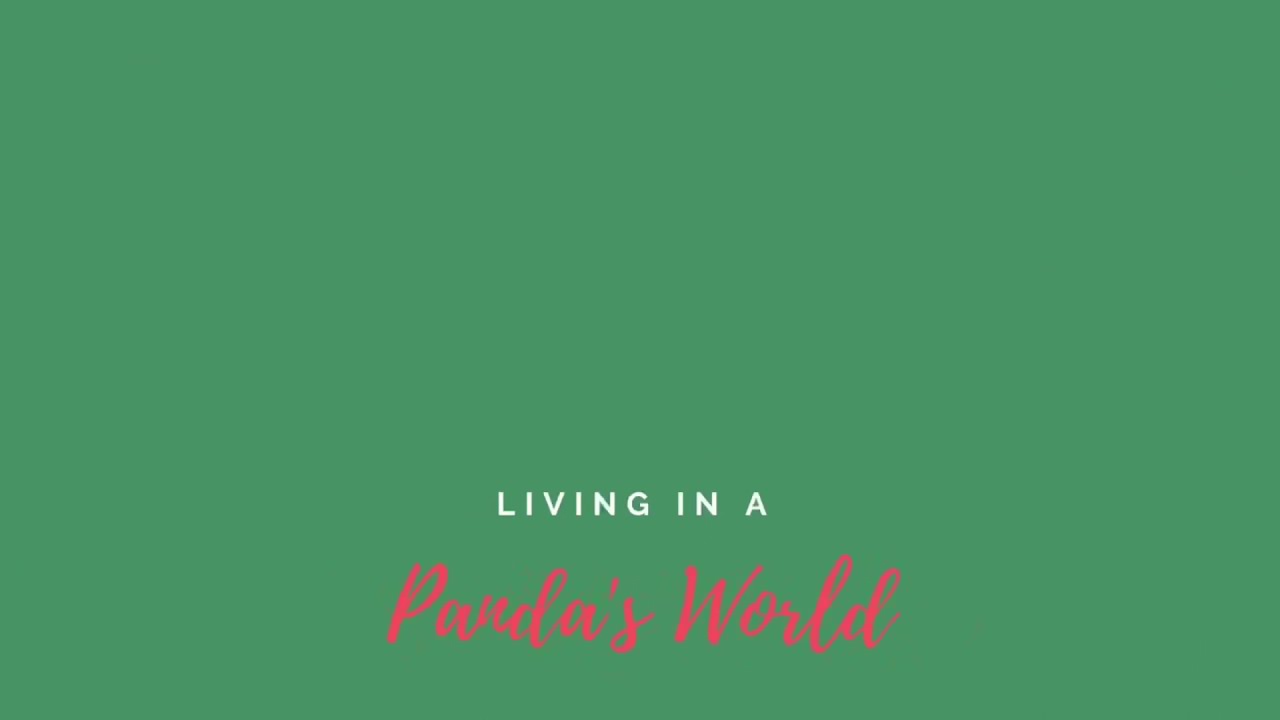The image features a solid green background, reminiscent of an evergreen or forest green shade. Dominating the center near the bottom are two rows of text. The top row reads "LIVING IN A" in all-uppercase, plain white sans-serif letters, making a stark contrast against the background. Directly below, in a larger, cursive font and in pink with a subtle black outline, it reads "PANDA'S WORLD." The cursive letters are interconnected, except for the "s" in "PANDA'S" and the "W" in "WORLD," which have slight separations. Despite the simplicity, the text is somewhat challenging to read due to reflections on the background and the cursive's shimmering quality. The overall color scheme with green, white, and pink hints at a festive or thematic context, possibly related to nature or an educational segment about pandas.